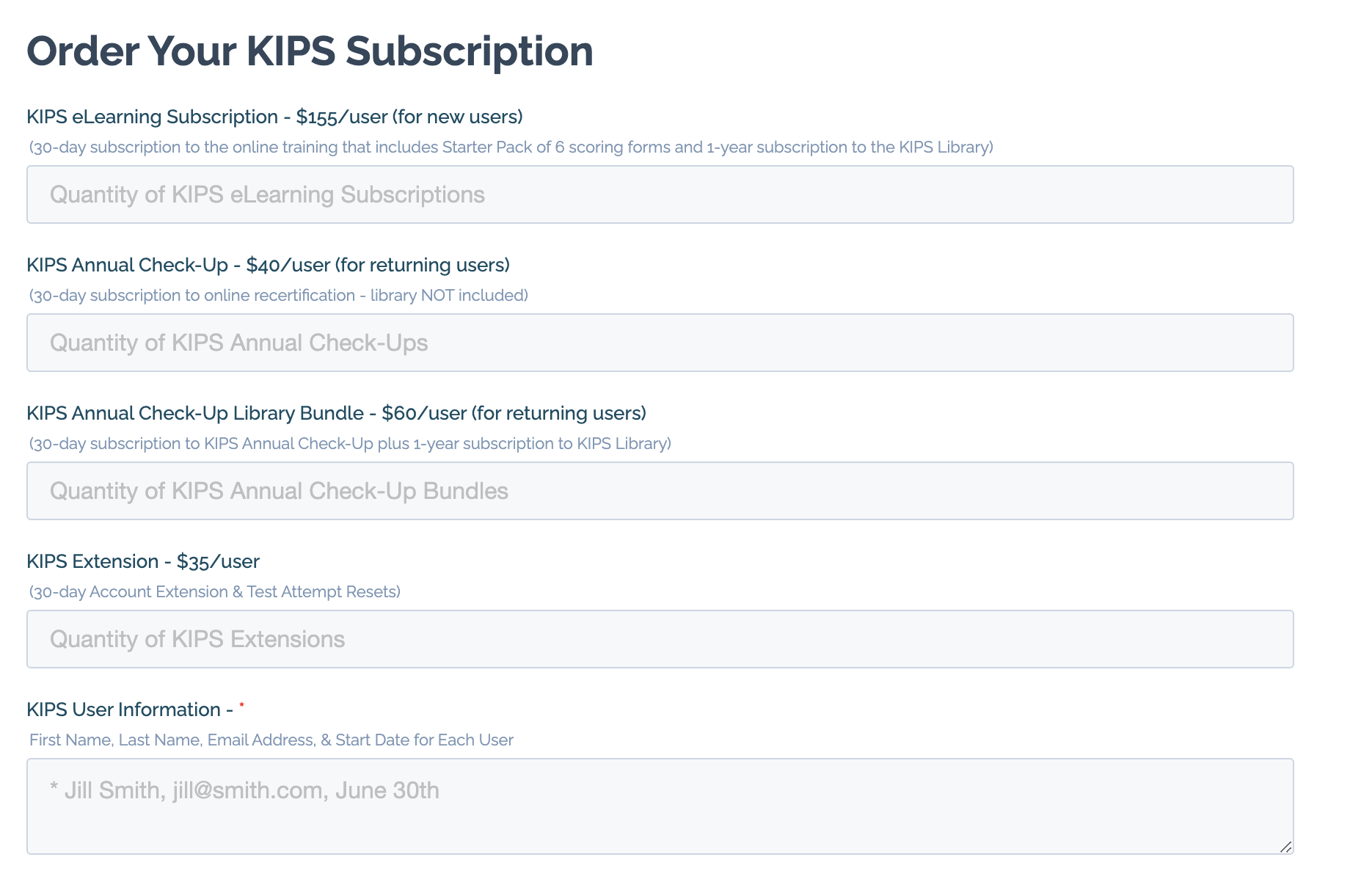This image displays a screenshot of a computer screen showcasing various subscription options for KIPS. At the top of the screen, in bold black print, there's a heading that reads "Order Your KIPS Subscription" followed by a subheading "KIPS eLearning Subscription." This subscription is priced at $155.00 per user for new users.

Beneath these headings, there are several sections with information and corresponding text boxes for user input. These sections feature titles in black text, and below each title, there are rectangular input boxes that have a subtle grayish-blue tint. Inside these boxes, the placeholder texts are rendered in gray.

Continuing down the list, there is a section titled "KIPS Annual Checkup," priced at $40.00 per user for returning users. Another option listed is the "KIPS Annual Checkup Library Bundle," which is priced at $60.00 per user for returning users.

Further down, there is a subscription option called "KIPS Extension," priced at $35.00 per user. Lastly, there is a section titled "KIPS User Information," which includes a text box where users can input their email address or any necessary information.